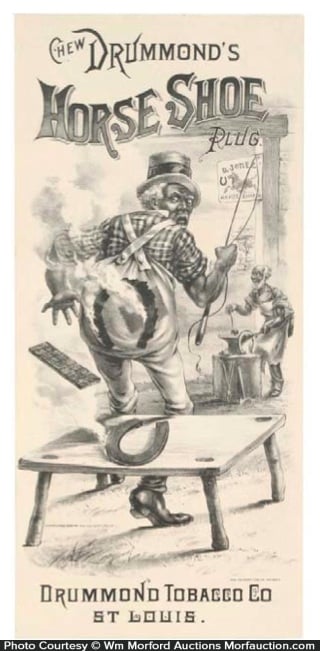This vintage-style advertisement poster, displayed on a cream-colored background, features the headline "Chew Drummond's Horseshoe Plug" in black font, with "horseshoe" written in a larger and ornate style. The bottom of the poster states "Drummond Tobacco Co. St. Louis." The central image depicts a humorous scene involving two African American men in a black and white illustration. 

In the foreground, a man stands with his back to the viewer, glancing over his shoulder. He is dressed in overalls over a flannel shirt and wears a top hat with a band around it. His pants show a seared pattern of a horseshoe, indicating he has just sat on a red-hot horseshoe, which is emitting smoke. The horseshoe itself lies on a small wooden table, also releasing smoke.

In the background, slightly to the right, another man, presumably a blacksmith, is engaged in his work. This man, wearing a large apron, is bald on the top of his head with visible lighter-colored hair at the back and a beard. He seems to be sharpening a tool or working on another horseshoe at an anvil.

At the very bottom of the poster, a black bar with white writing notes, "Photo courtesy W.M. Morford Auctions, morfordauction.com." This image embodies the rustic charm and advertising style of yesteryears while delivering a comedic narrative.